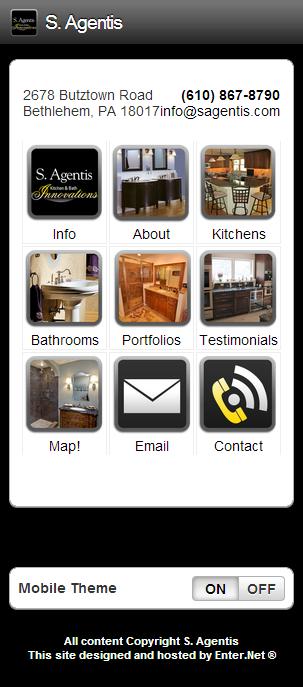The screenshot depicts a mobile screen with a predominantly black background and a central white, rounded rectangle displaying the address "2678 Butztown Road, Bethlehem, PA 18017" and a phone number "610-867-8790." Below the address, there's an email, info@sagentis.com. Located at the top left corner, the name "S. Agentis" is prominently displayed. The central feature of the screen includes a grid of nine buttons arranged in three rows and columns, each with an associated icon and label. The buttons are labeled: Info, About, Kitchens, Bathrooms, Portfolios, Testimonials, Map, Email, and Contact. At the bottom of the screen, there is a toggle switch labeled "Mobile Theme," which is set to on. The footer of the screen displays the text "All content copyright S. Agentis. This site designed and hosted by Enter.net."